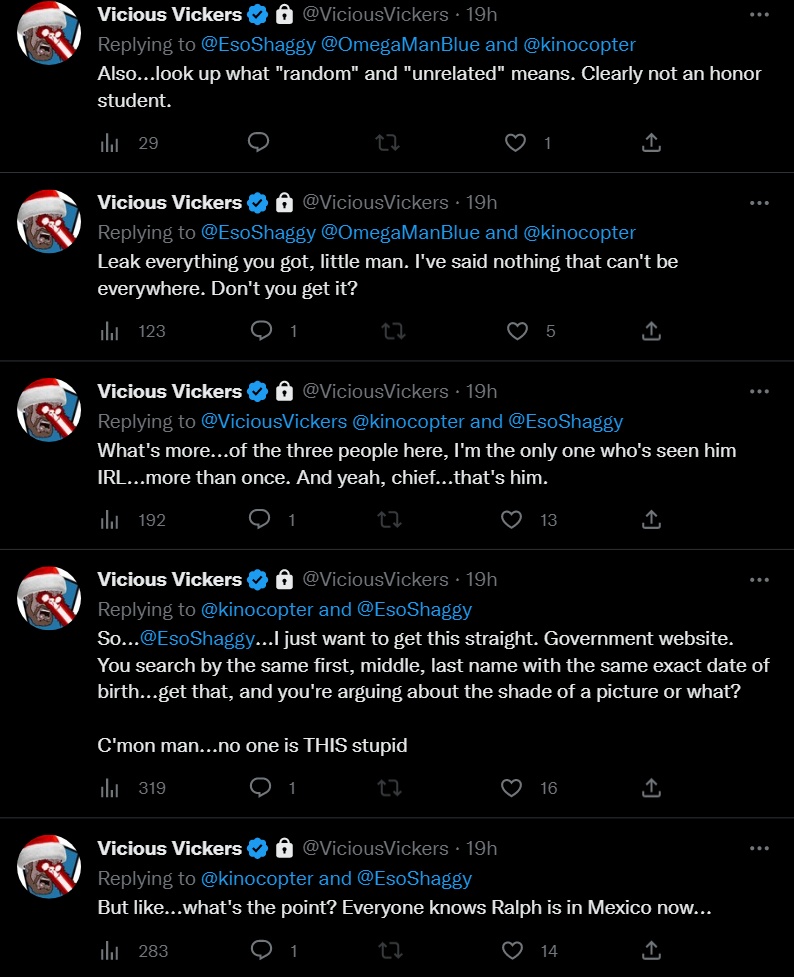A detailed caption for the image could be:

"This image is a screenshot of several Twitter posts made by a user named 'Vicious Vickers'. The background of the image is black. Each tweet comes from the same account and features a profile picture of a man with a beard wearing a Santa hat, shooting rays out of his eyes towards the bottom right. His profile picture is set against a blue square, with minimal white borders on the top, left, and right sides.

To the right of the profile picture, the user's name 'Vicious Vickers' is bolded in white. Next to his name, there is a blue circle bearing a white or black check mark, indicating a verification status, and a white lock icon. Below his name, in gray text, it displays '@ViciousVickers' followed by '19h,' indicating the posts were made 19 hours ago.

Each tweet by Vicious Vickers is a reply to different users: '@EchoSoShaggy,' '@OmegaManBlue,' and '@KinoCopter.' These replies are visibly consistent across the posts.

Each tweet also contains various engagement metrics:
1. The first post shows '29 views,' along with icons for comments, shares, likes (with one like), and downloads.
2. The second post has '192 views,' one comment, and 13 likes.
3. The third post records '319 views,' one comment, and 16 likes.
4. The fourth and last post shows '283 views,' one comment, and 14 likes.

In the top right corner of each tweet, there are gray ellipses, hinting at more options available for each post."